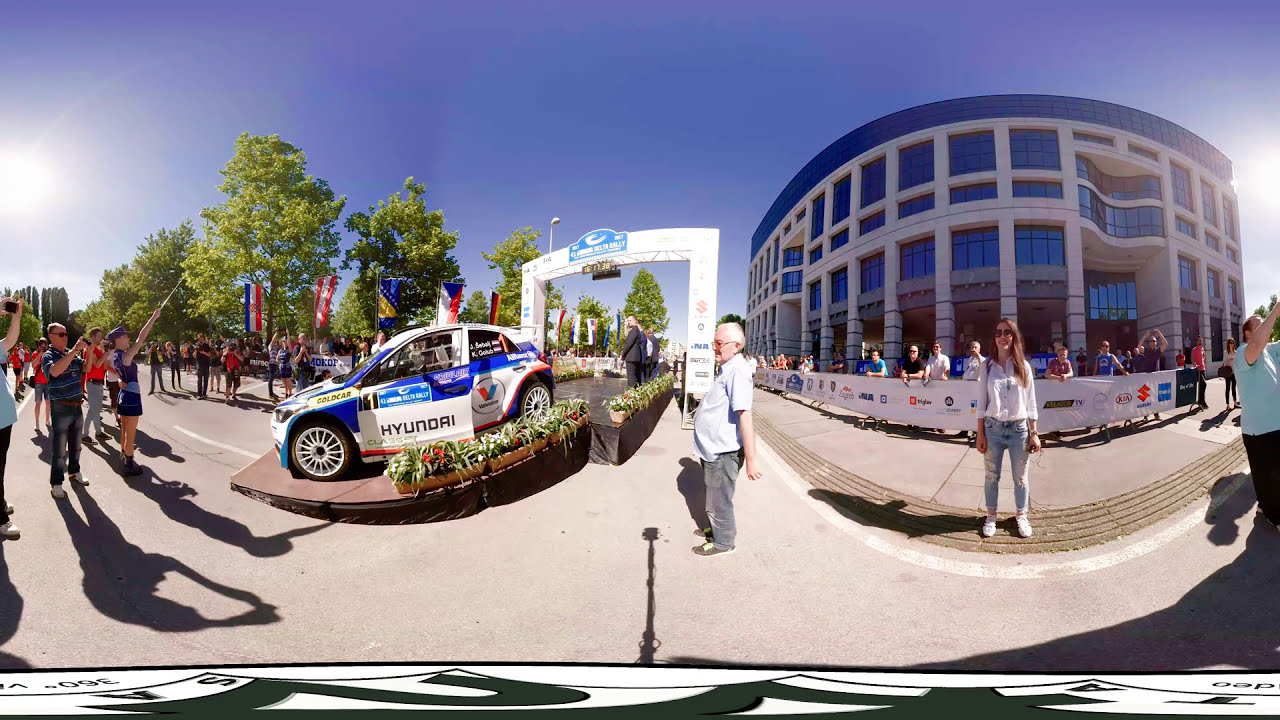The image is a wide rectangular panorama capturing a lively, outdoor celebratory event in an urban environment. On the left side, a gray paved road curves from the middle to the left, bordered by a gathering of people taking pictures and observing the scene. Prominently displayed on a plant-covered brown platform ramp is a white and blue Hyundai race car, with "Hyundai" written in black letters on the driver's door. Behind the car are several hanging flags and a backdrop of very tall light green trees.

Dominating the right side of the image, there's a large white and blue mid-sized building with giant blue windows and a blue roof, adding to the vibrant color palette of red, white, blue, and green. A woman stands prominently in front of this building. The bright blue sky transitions to white at the edges, emphasizing the natural light that bathes the entire setting, giving it a vivid and lively atmosphere. The press appears to be present, highlighting the car under a canopy or arch, indicating the event's importance.